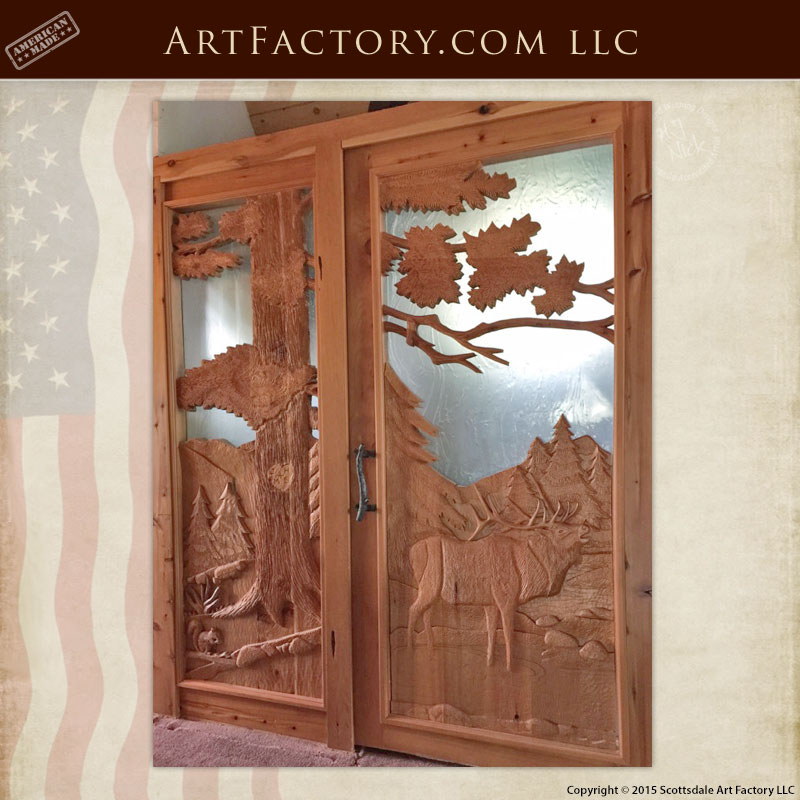The image features an intricate, American-made wooden door frame, intricately carved with outdoor scenes. The door, made by Artfactory.com LLC, depicts a majestic moose or caribou standing in water, its large antlers arching back over its head towards its mid-back. Surrounding this centerpiece are detailed carvings of both deciduous and pine trees, with a mountain visible in the background. A tall tree occupies the left panel, accompanied by smaller trees and a squirrel. The top of the door features glasswork and wood overlay with tree branches and leaves, while a black handle adorns the door. Above the door, a brown banner with cream-colored writing reads "Artfactory.com LLC, American Made." Additionally, a faint image of a vertical American flag can be seen on the left side. The bottom corner of the image notes "Copyright 2015, Scottsdale Art Factory LLC."